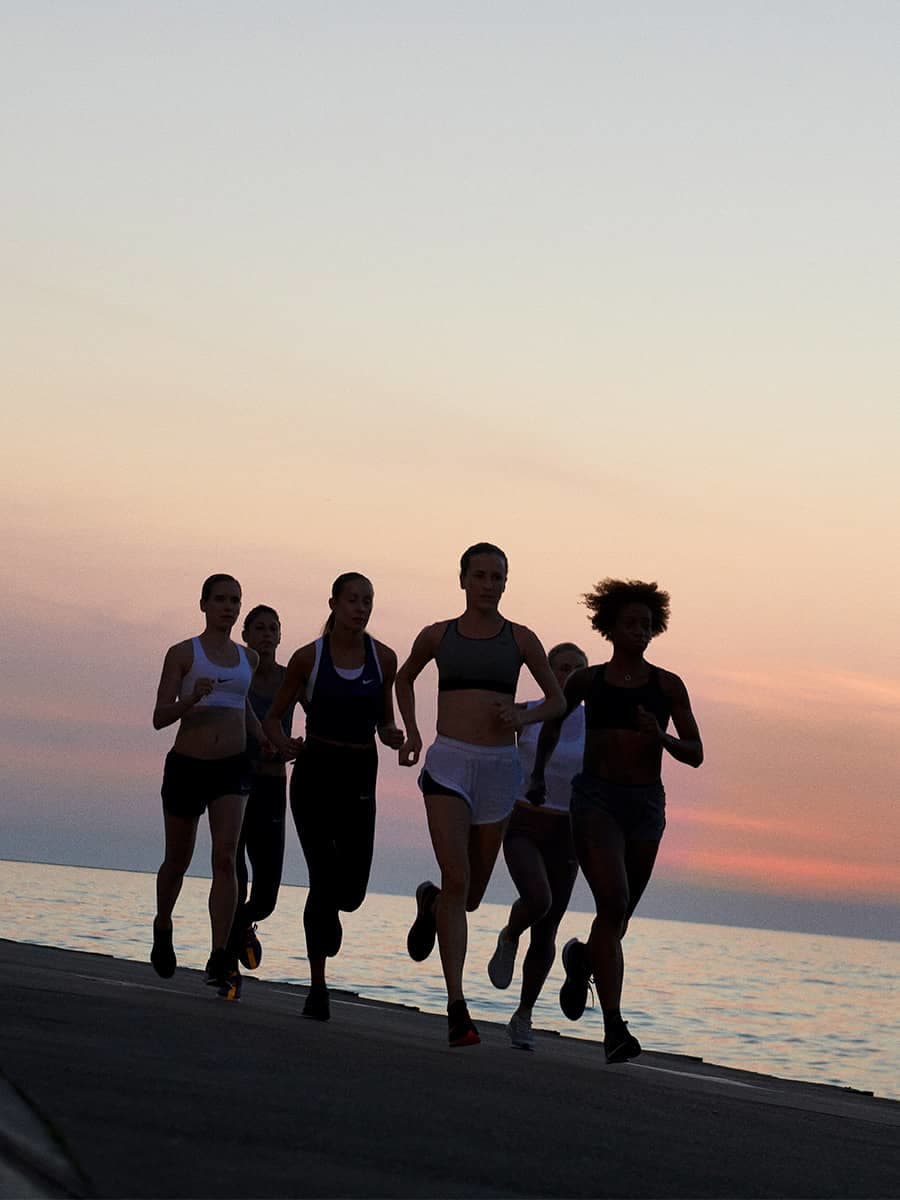The photo captures a group of six athletes, mainly women, jogging near a shoreline during a captivating sunset. The scene is bathed in the purplish and gray hues of dusk, with the ocean and clouds forming a picturesque background. The runners, clad in short shorts, sports bras, and some in bodysuits, are moving along a concrete trail that slightly slopes downhill from the left to the right side of the image. Most of the women are either Black or Hispanic, with dark hair pulled back into ponytails, while one woman has short, free-flowing hair. Reflectors are visible on a few of their shoes, adding a subtle glow to their strides. The pack includes five women and possibly one man who trails behind. The serene yet dynamic moment is encapsulated without any text, highlighting the harmony of athleticism and nature.